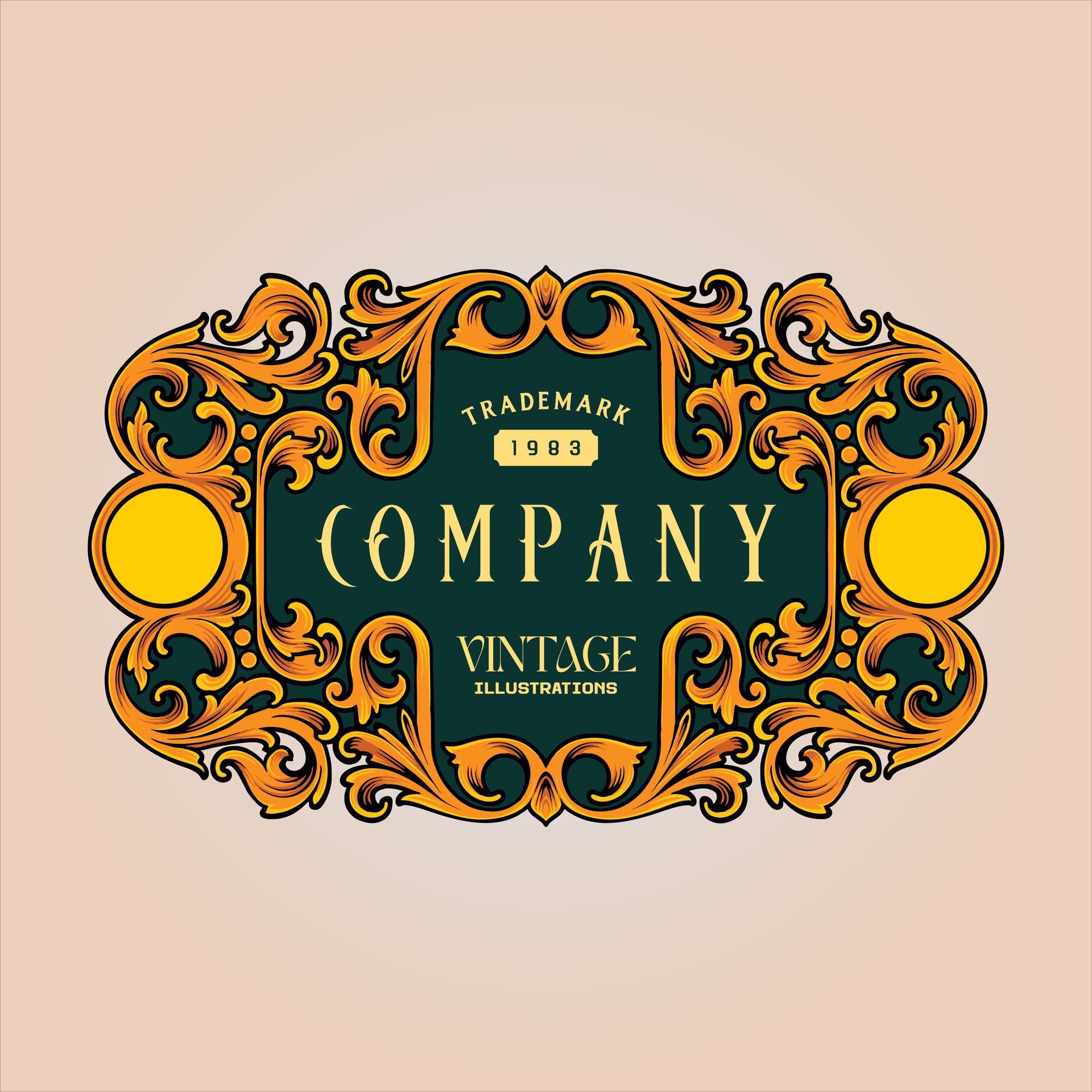The image displays a company's logo set against a backdrop that appears to be a muted green color, possibly with hints of grey or blue. The foreground is adorned with intricate golden yellow lines and scrolls, resembling elegant, almost royal decorations that form a border around the central rectangular design. On either side of this border, there are prominent yellow circles. Within the frame, the text "Trademark 1983" is prominently featured at the top in large, ornate white letters. Below this, in a similar decorative font, the word "Company" is displayed, followed by the phrase "Vintage Illustrations" in another stylish script. The combination of gold ornamental lines, yellow circles, and the sophisticated lettering creates a classic and timeless appearance, reinforcing the company's vintage and artistic branding.